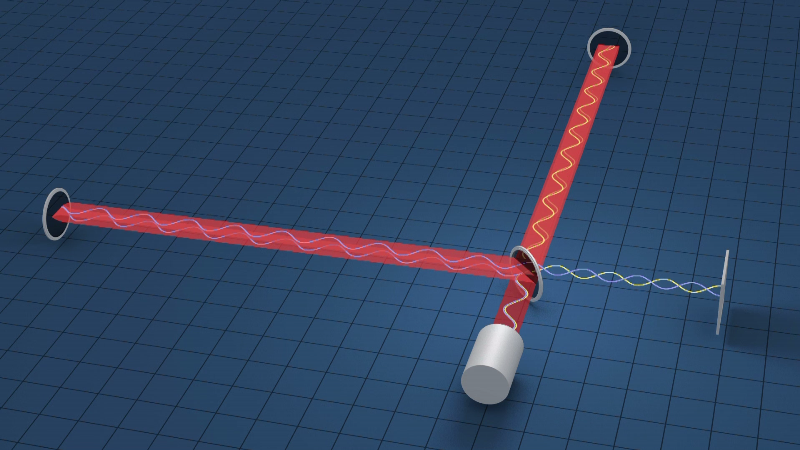The image depicts a detailed and intricate diagram set against a blue and dark blue squared grid background, outlined in black, creating a checker pattern. At its core, the central feature is a complex contraption composed of several interconnected components. Dominantly, there are two red beams. The first red beam runs horizontally from a black circle with a silver outline, ending in a metal squiggly shape at the contraption’s flat base. From the base, a silver cylindrical form rises, transitioning into a second red beam adorned with undulating yellow patterns. This second red beam extends vertically to connect with a middle black circle, also outlined in silver, resembling a portal. On the right, this red beam produces a blue and yellow DNA-like helix, which then enters a square shape. Overall, this diagram appears to illustrate a process involving beams and reflections, possibly signifying a scientific or technological phenomenon where elements interact and reflect within a structured grid.